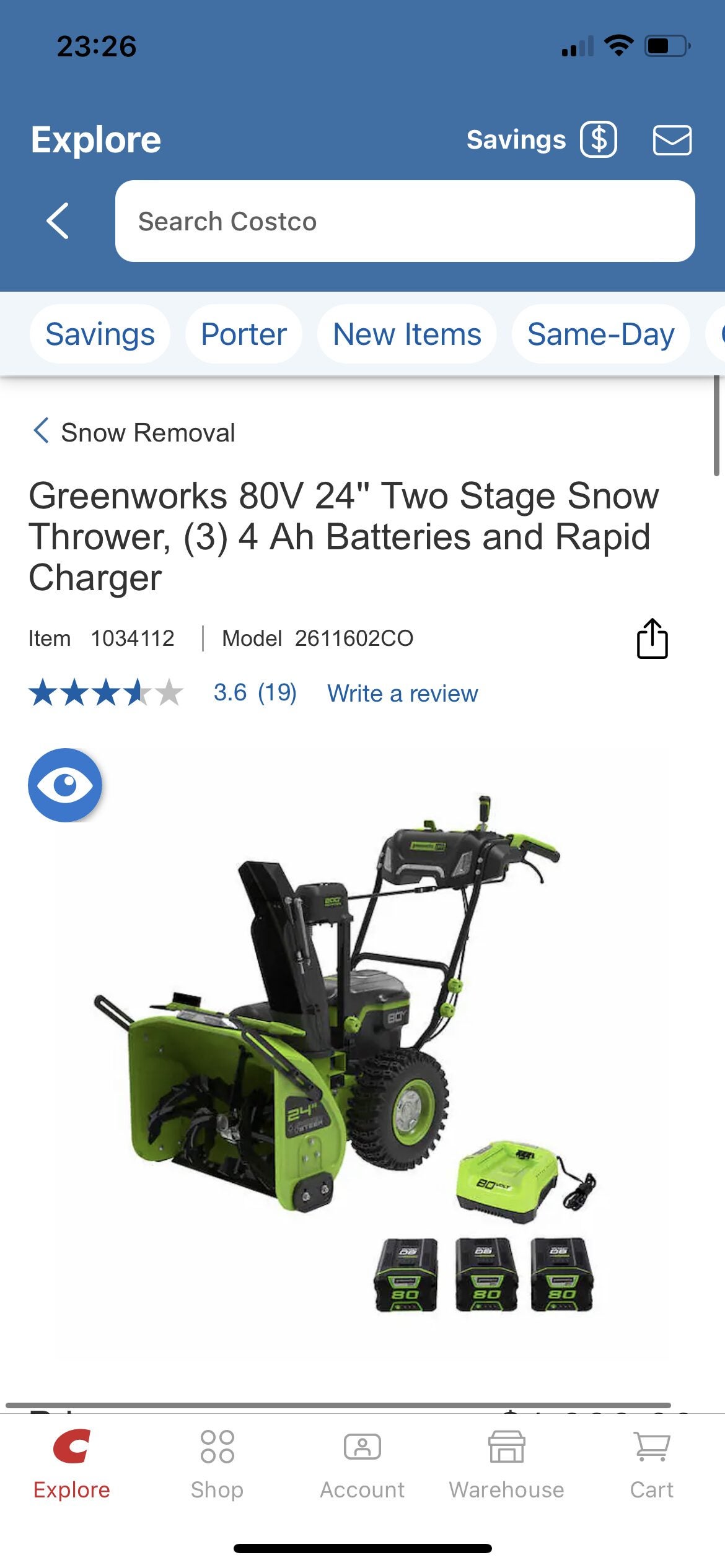A screenshot from a mobile device displays the Costco website or app, showcasing a product detail page for the Greenworks 80V 24-inch Two-Stage Snow Thrower. This electric snow thrower, primarily green and black, includes three 4.0 Ah batteries and a rapid charger, making it convenient for users to swap out batteries as needed. The interface features a prominent explorer bar at the top and a search bar. Notable details about the product include a 3.6-star rating out of 5 based on 19 reviews. While the background is largely white, the iconic Costco blue is visible at the top of the page. Navigation tabs at the bottom of the screen include options for Explore, Shop, Account, Warehouse, and Cart. Notably, the price of the snow thrower isn't visible in the screenshot.